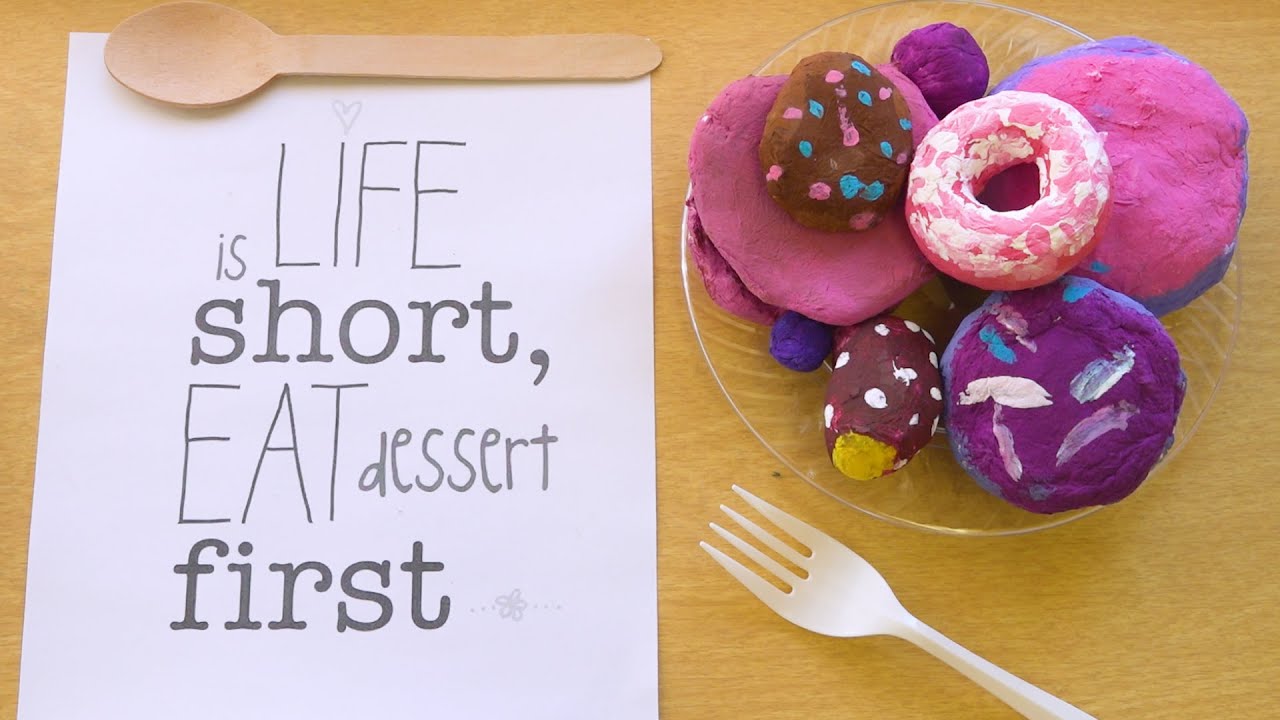The image features a soft tan background, likely a wooden table, adorned with a variety of elements. A white piece of paper on the left side bears an inspiring message in various fonts and sizes: "LIFE is short, eat dessert first." The word "LIFE" is emphasized in large capital letters with a heart dotting the 'i', while "short" and "first" are in a typewriter font and "dessert" is in a handwritten style. At the top of the page lies a wooden spoon, and a white plastic fork is positioned on the bottom right.

Beside the paper, an assortment of painted rocks resembling donuts and cookies spreads out. These rocks vary in size and shape, some flat, some round, and some even featuring a hole in the center. The delicately painted designs include pink cookies with purple edges, blue cookies with purple frosting accents, and donuts adorned with white icing or decorated with pink and blue dots. Accompanying these treats is a glass dish with a patterned edge, adding a final touch to this sweet display.